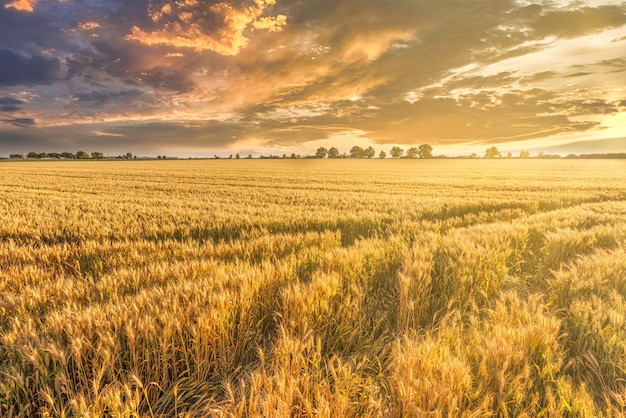The image captures an expansive outdoor scene dominated by seemingly endless fields of golden wheat, stretching as far as the eye can see. Acres upon acres of wheat, its furrows hinting at pathways walked through, occupy the majority of the image, meeting a distant horizon lined with tall green trees. Above this vast wheat landscape, the sky provides a dramatic contrast, featuring a gradient of clouds ranging from dark blue and gray on the left to orange and gray in the center, and gray and white on the right. The overall golden hue of the wheat suggests a sunset, casting a warm glow over the entire scene and enhancing the rich textures and colors of both the crops and the sky.